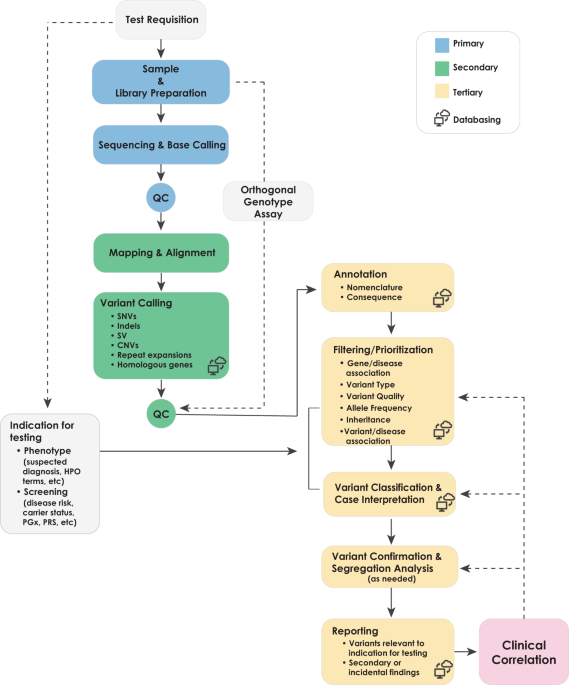This illustration is a detailed medical flowchart that outlines the multistep process of genomic testing and data interpretation. The diagram starts from the top-left with a light gray rounded rectangle labeled “Test Requisition.” From there, an arrow points downward to a blue rounded rectangle named "Sample and Library Preparation," followed by another blue rectangle titled "Sequencing and Base Calling." Next, a blue circle labeled "QC" connects to a green rectangle named "Mapping and Alignment." 

The flow continues to another green rectangle called "Variant Calling," which lists specific variant types like SNVs, indels, SV, CNVs, repeat expansions, and homologous genes. This is followed by another green circle for "QC". From the green QC, an arrow leads to a yellow rectangle on the right marked "Annotation" with sub-bullets indicating nomenclature and consequence. 

The next stage down within yellow rectangles includes "Filtering and Prioritization" with bullet points such as gene-disease association, variant type, variant quality, allele frequency, inheritance, and variant-disease association. Following this, another yellow rectangle reads "Variant Classification and Case Interpretation." Subsequent steps involve a yellow rectangle titled "Variant Confirmation and Segregation Analysis (as needed)" and a final yellow rectangle labeled "Reporting: Variants Relevant to Indication for Testing, Secondary or Incidental Findings." The flowchart concludes at the bottom right with a pink rectangle named "Clinical Correlation," which links back to the preceding yellow rectangles.

Additionally, on the left, a light gray rectangle tagged "Indication for Testing" connects to "Test Requisition" via a dashed line. This includes details such as phenotype, suspected diagnosis, HPO terms, disease risk, carrier status, PGX, PRS, etc. The diagram is supported by a legend in the top right, which explains the color coding: blue for primary processes, green for secondary, yellow for tertiary, and an icon system representing databasing activities.